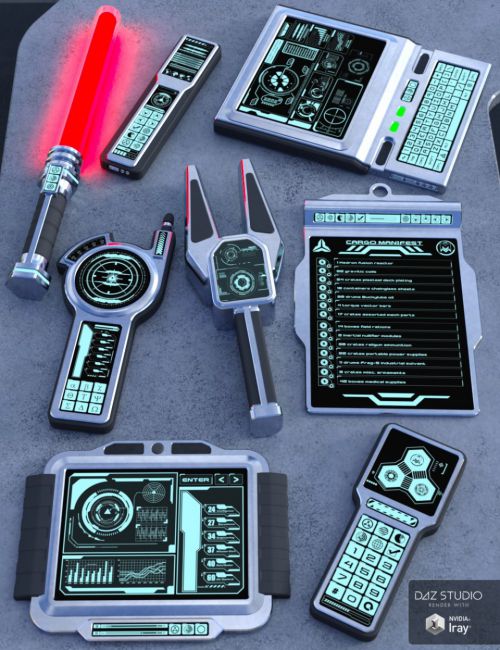The image showcases a collection of futuristic, handheld technological devices arranged on a gray background. The devices share a consistent aesthetic, primarily in shades of steel blue, black, and white, featuring a light blue coating. 

On the top left, there is a miniature lightsaber with a glowing red blade. To its right, near the center, is a long, vertical rectangular device resembling a phone. Adjacent to this, there is a flat computer with a blue digital keyboard and a black screen displaying blue symbols and signals. 

Below this screen is a digital clipboard with a black screen. In the center, there's an object resembling an airport security monitor or scanner. On the far left in the middle, there's a circular device that appears to be a detector of some kind. 

At the bottom left, a rectangular tablet with similar signals and symbols is situated. To its right, a slender, rectangular phone-like device is placed. 

Other items mentioned include devices that resemble GPS systems, remote controls, and possible iPad-like gadgets. The entire arrangement appears to be a conceptual display for a kit of advanced security or spy gear, possibly for a game or show, and is labeled as a creation by Dayz Studio, NVIDIA, and IRAE.